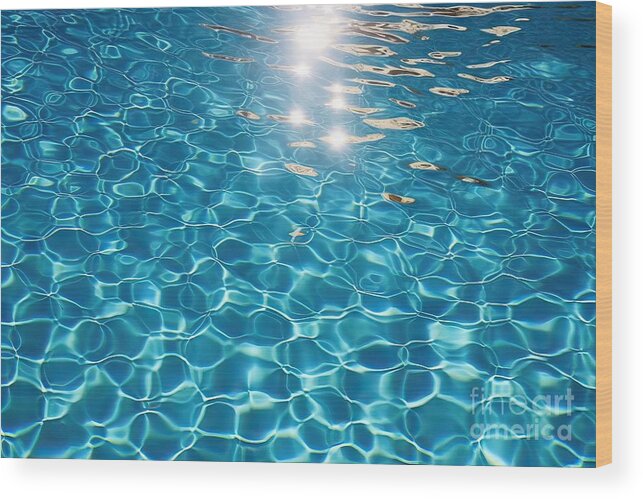This photograph captures a vivid close-up of sparkling blue water, likely from a swimming pool or a clear ocean with white sand. The water is crystal clear, shimmering under bright sunlight, which pours down the center top of the image and creates bright white reflections and interlocking ripples. These ripples form irregularly-shaped, yet repetitive, patterns of tiny blue and white circles across the entire scene. The right side of the photograph features a thin, tan-colored outline, adding depth to the composition. In the bottom right-hand corner, a watermark reads "Fine Art America" in distinct white fonts, emphasizing the artistic nature of the photograph. This image was taken during the day, evident from the natural sunlight glistening on the water, producing an enchanting interplay of light and shadows.